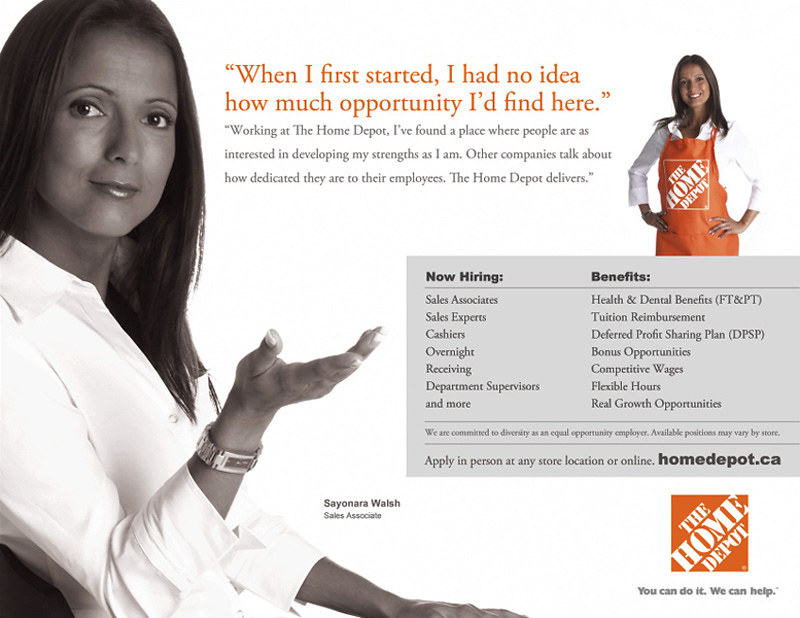The image is a hiring advertisement for The Home Depot. The background is primarily white, featuring a central message and photos highlighting an employee's experience and opportunities available at the company. On the left side, there is a woman with long dark hair, dressed in a white button-down collared shirt, looking directly at the camera with her right hand raised. The text next to her reads: "When I first started, I had no idea how much opportunity I'd find here. Working at The Home Depot, I found a place where people are as interested in developing my strengths as I am. Other companies talk about how dedicated they are to their employees. The Home Depot delivers."

To the right of this paragraph, there is another photograph of likely the same woman, now wearing a white button-down shirt paired with an orange Home Depot apron. Below this image, the text reads "Now Hiring," followed by a list of open positions including sales associates, cashiers, overnight receiving, and department supervisors. Adjacent to this, another section outlines the benefits offered by the company such as health and dental insurance, tuition reimbursement, a deferred profit-sharing plan, bonus opportunities, competitive wages, flexible hours, and real growth opportunities.

At the bottom of the advertisement, there's the Home Depot logo accompanied by their slogan: "You can do it. We can help." Furthermore, it mentions the woman's name, Sayonara Walsh, identifying her as a sales associate. This detailed portrayal aims to attract potential employees by showcasing a positive and supportive work environment.